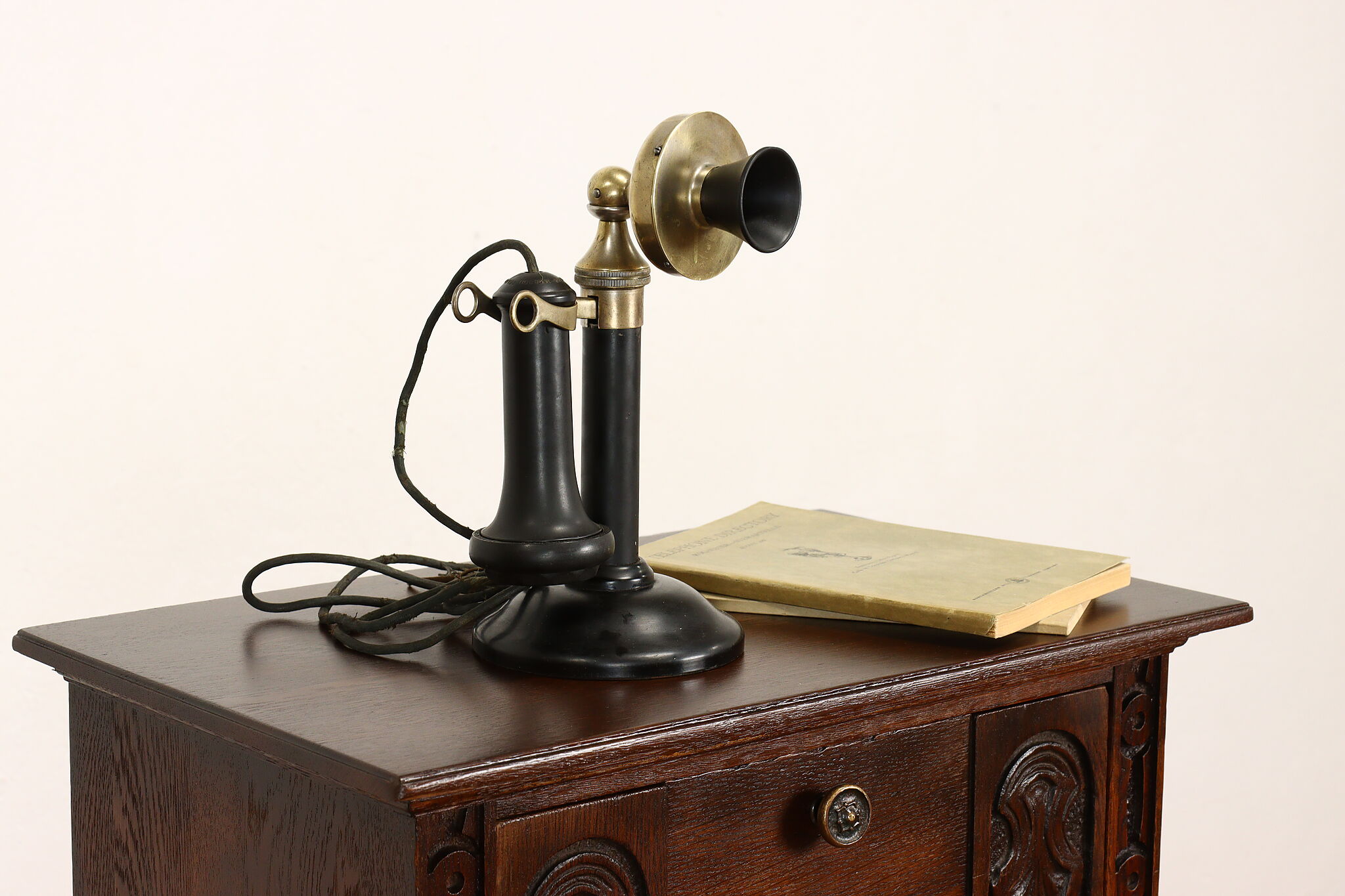This photograph captures a close-up of a vintage telephone displayed on a dark, intricately designed wooden stand with a small drawer featuring a knob. The telephone, possibly one of the first models ever invented, is composed of two parts: a brass speaker with a long tube and flared base, and a separate, corded listening piece hanging off to the side. The telephone showcases a classic black and golden color scheme. Situated next to the telephone on the stand are two old books or notepads with light yellowed pages, possibly vintage phone books, though the text on them is too faded to read. The background of the image is a plain cream white, which accentuates the detailed and nostalgic elements of the telephone and furniture.